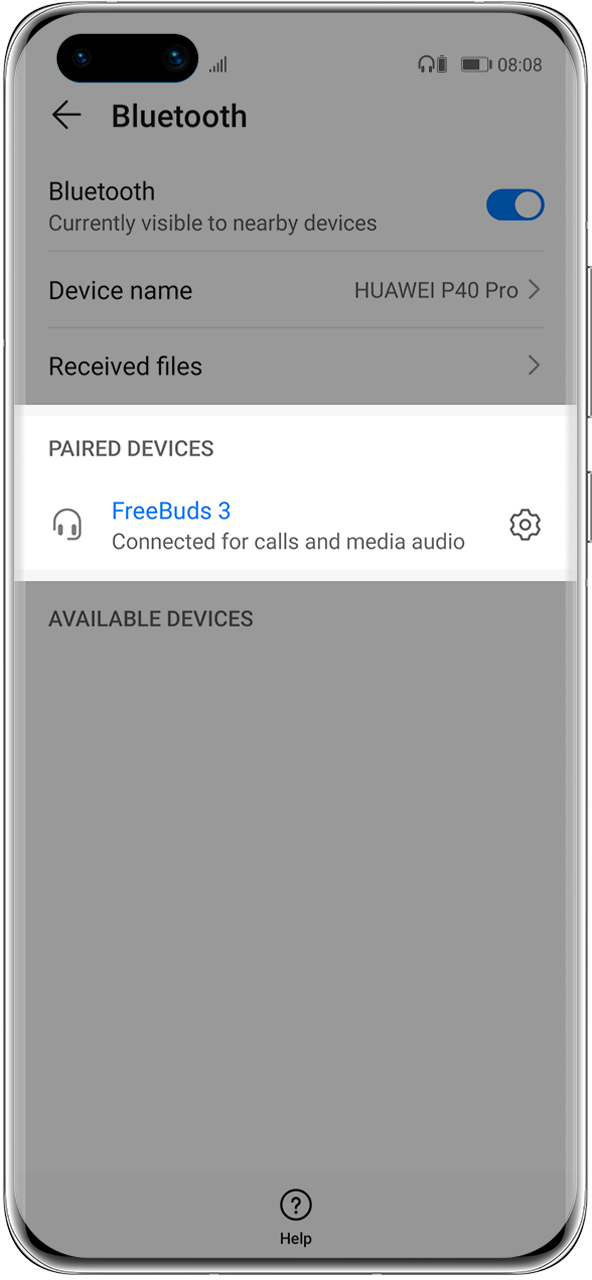The image is vertically rectangular, showcasing the screen of a Huawei P40 Pro smartphone in the Bluetooth settings menu. The phone's display features a thin frame around the edges, and the screen itself is visible. At the top of the settings, the Bluetooth toggle is switched on, indicating that the device is currently discoverable to nearby devices.

Beneath the toggle, the device name "HUA-WEI P40 Pro" is displayed prominently. There is also an option for "Received files". Below this, a white horizontal rectangular section stands out against the otherwise gray background, labeled "Paired devices." Within this section, a device named "FreeBuds 3" is listed as connected for calls and media audio.

Resuming to the gray background, the screen lists "Available devices," indicative of other Bluetooth devices visible for pairing. At the very bottom of the screen, there is a question mark icon with the label "Help" beneath it.

Additionally, as this is an image of the phone itself, the front camera is visible in the upper left corner of the frame. The status bar displays the headphone icon, battery icon, and the current time, which is 8:08 AM.